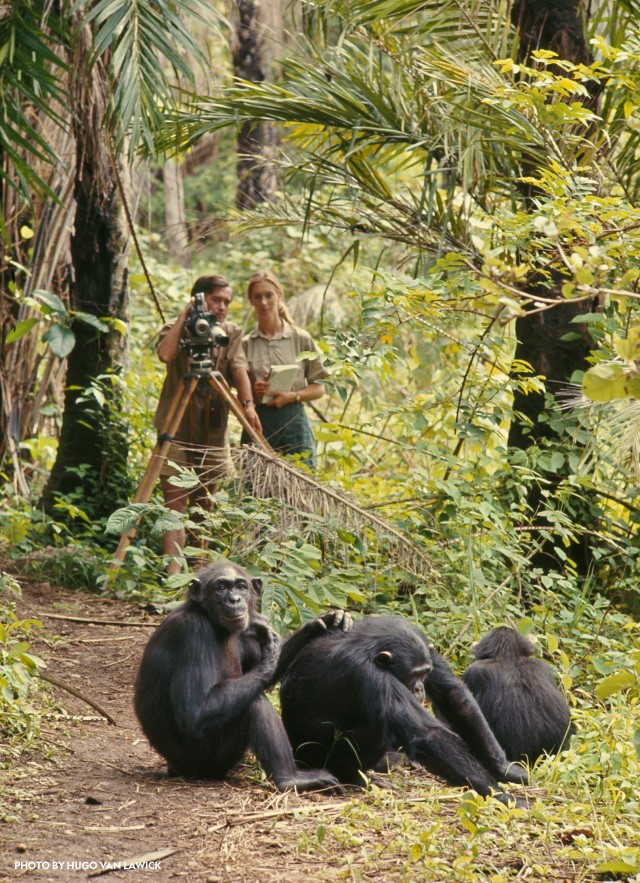In this captivating photograph set in a dense jungle, three chimpanzees are prominently featured in the foreground, sitting on a mix of dirt ground and vibrant green leaves. On the left, an adult female chimpanzee gazes directly at the camera while placing her hand on the back of the middle chimpanzee, as if scratching or grooming it. The middle chimpanzee, an adult male, is hunched over with its arms stretched forward and resting on the ground, eyes downcast. On the right, a smaller, adolescent chimpanzee sits with its back turned to the camera, appearing to look toward the two humans in the background. Behind the chimpanzees, a man stands beside a wooden tripod-mounted camera, while a woman beside him holds a notebook. Both are focused intently on the chimpanzees. The scene is surrounded by lush, leafy trees, adding to the sense of a natural, wild environment.